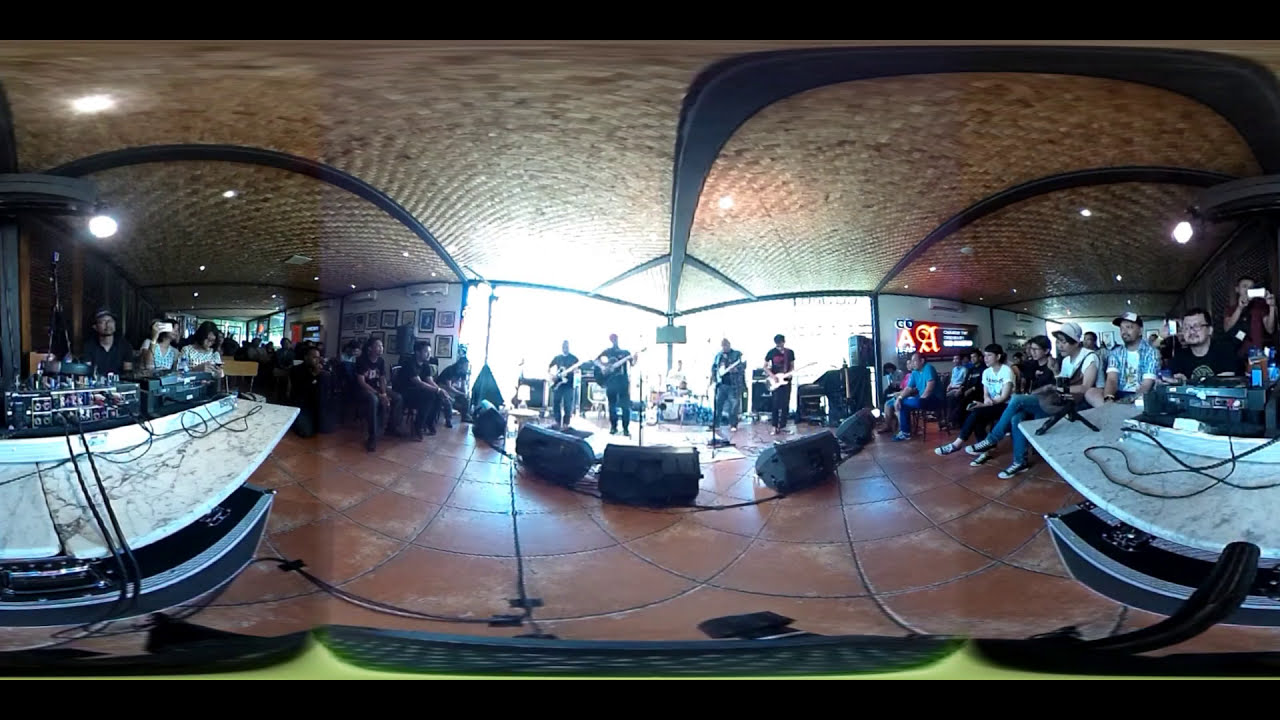The image captures a dynamic scene within a bar or hall where a band is performing. The band consists of five male members, with four guitarists positioned at the front—two on the left and two on the right—all dressed in dark clothing. At the center behind them, the drummer is visible, encircled by a ring of black speakers that amplify their music. The overall image has a distorted, almost fisheye effect, causing the left and right sides of the scene to curve inward, giving it a surreal appearance. On both sides of the venue, audience members, both male and female, are seated and focused on the performance. Each guitarist has a speaker stand beside them, and tables laden with PA equipment, including amplifiers and sound systems, are visible, ensuring the sound quality is maintained. The dance floor at the front is spacious, and the ceiling features a unique cork-like texture with black edging. An illuminated sign reading "Go A" in an orange-reddish hue is displayed prominently at the back of the stage. The floor is paved with reddish clay-colored tiles, complementing the warm, ambient atmosphere of the venue.